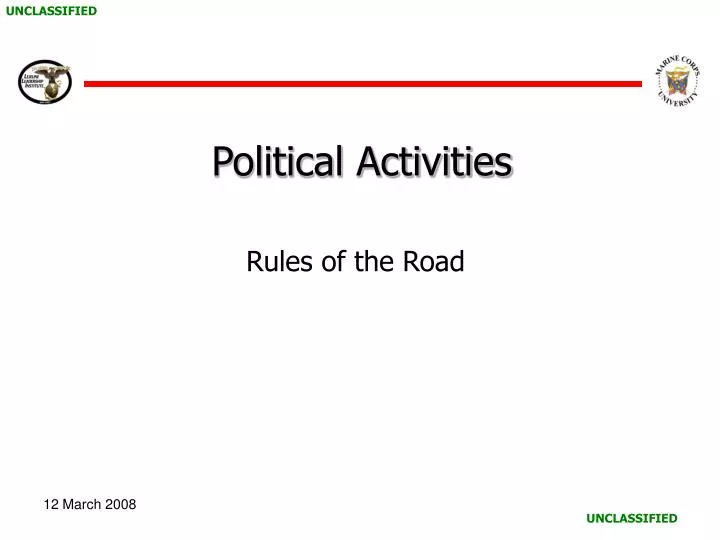The image is likely part of a government presentation slide titled "Political Activities, Rules of the Road." The central text features "Political Activities" in a bold, dark black font, larger than the subtitle "Rules of the Road." The top and bottom corners of the slide, which has a plain white background, have the word "UNCLASSIFIED" in green, uppercase letters. A red line horizontally divides the upper part of the slide, flanked by two circular emblems. The emblem on the left depicts an eagle with outstretched wings and is linked to a U.S. government department, though its accompanying text is too blurry to read. The emblem on the right features an eagle perched on a globe, encircled by the words "Marine Corps University". The date "12 March 2008," is printed in black in the bottom left corner.